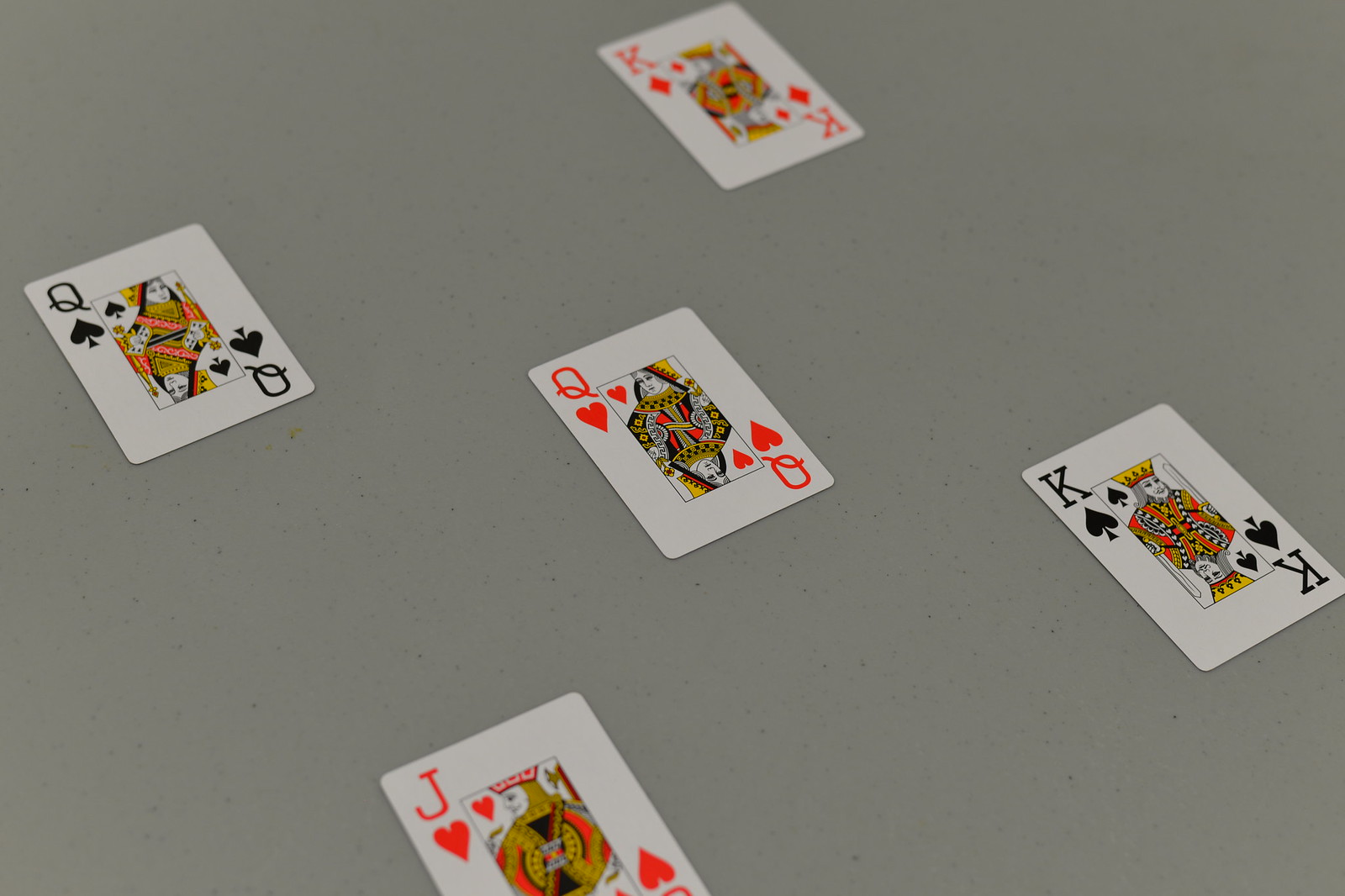This photograph captures a set of five playing cards turned face up on a sleek, gray speckled playing surface. The surface itself has a professional, non-reflective finish with black speckles interspersed across a neutral gray background, indicating it's designed specifically for gaming purposes due to its smooth and flat nature. The cards appear to be in pristine condition. The image composition shows a narrow focal range, which brings the center three cards into sharp focus, while the top and bottom cards remain slightly blurred. From what is visible, the cards depict a King of Diamonds at the top, the Queen of Spades on the left, the Queen of Hearts at the center, the King of Spades at the bottom right, and the Jack of Hearts at the bottom center. The aesthetic arrangement and selective focus highlight the intricate details of the playing cards against the refined backdrop.